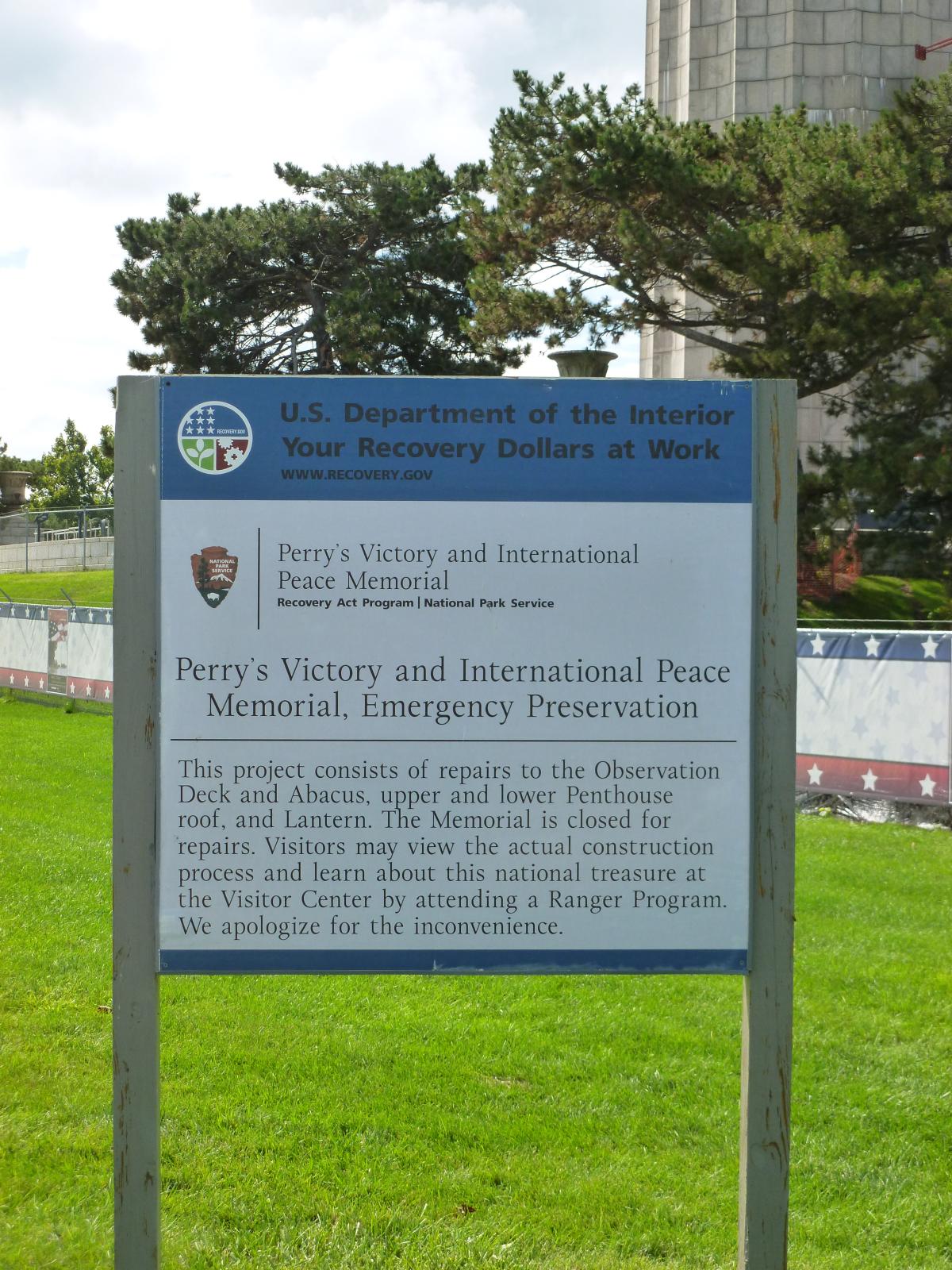The image, captured during a clear, sunny day with blue skies and clouds, depicts an outdoor scene dominated by a prominent sign displayed on a grassy field. The sign, with a blue header taking up about a quarter of its area, reads "U.S. Department of the Interior, Your Recovery Dollars at Work," alongside a logo featuring stars from the American flag, a plant with three leaves, and interlocking gears. Below the blue header, in black text, it states "Perry's Victory and International Peace Memorial" and "Perry's Victory and International Peace Memorial Emergency Preservation." A detailed paragraph beneath explains the project: "This project consists of repairs to the observation deck and abacus, upper and lower penthouse roof, and lantern. The memorial is closed for repairs. Visitors may view the actual construction process and learn about the national treasure at the visitor center by attending a ranger program. We apologize for the inconvenience."

In the background, there is a roundish water tower building to the right, partially obscured by trees. A wall and a fence, akin to those around sports stadiums, stretch along the lower part of the scene. This setup directs attention to the significant restoration efforts underway at the historic site.